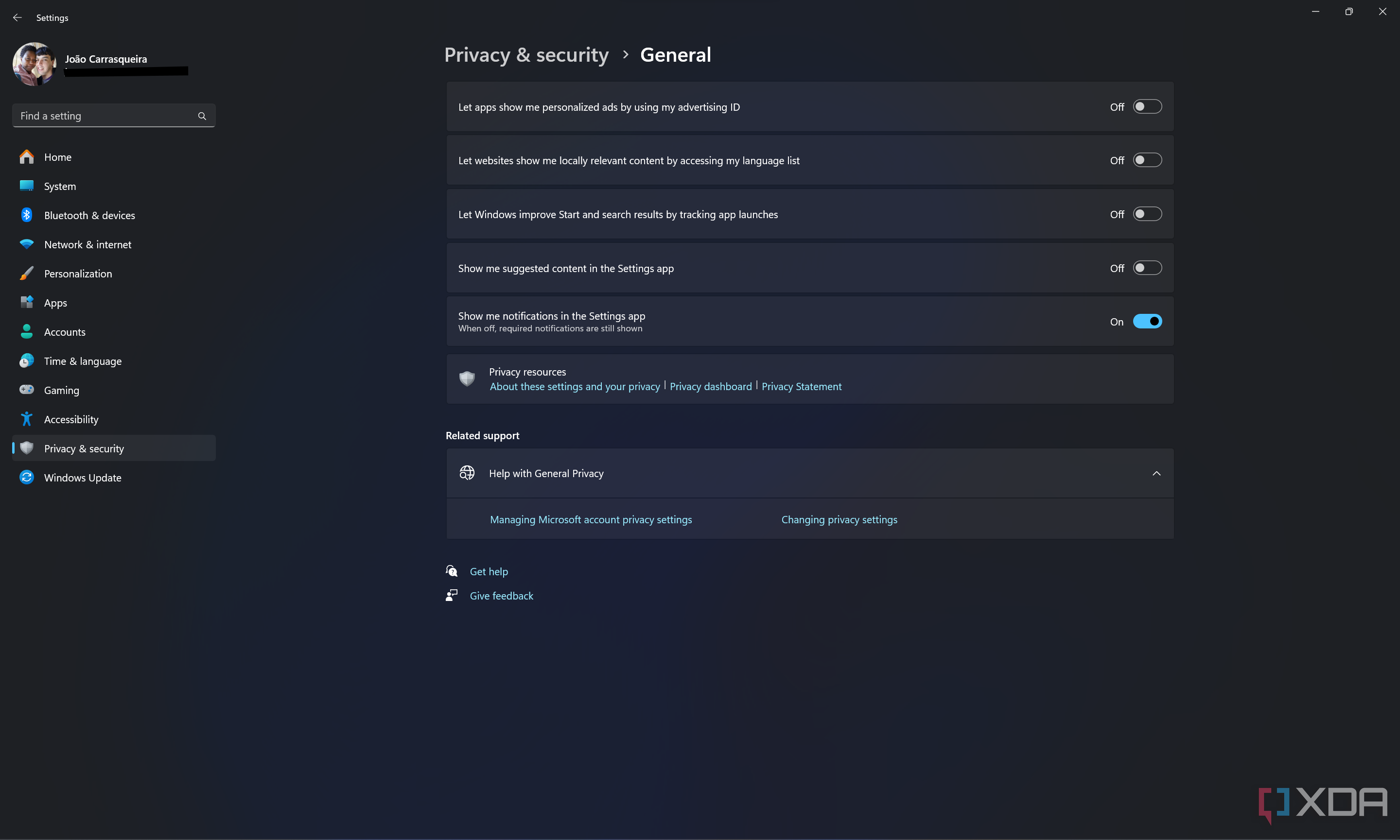The image shows a computer screen displaying the Windows Settings interface against a black background. In the top right corner, the minimize, maximize, and close (X) buttons are visible. On the top left corner, there is a profile picture, although the associated name is too small and blurry to read. 

The left sidebar includes a search box labeled "Find a setting" and a list of menu options:
- Home
- System
- Bluetooth & Devices
- Network & Internet
- Personalization
- Apps
- Accounts
- Time & Language
- Gaming
- Accessibility
- Privacy & Security
- Windows Update

The main section of the screen highlights the "Privacy & Security" settings, specifically the "General" category. The following toggles are visible:
- "Let apps show me personalized ads by tracking app launches" (turned off)
- "Let websites show me locally relevant content by accessing my language list" (turned off)
- "Let Windows improve Start and search results by tracking app launches" (turned off)
- "Show me suggested content in the Settings app"